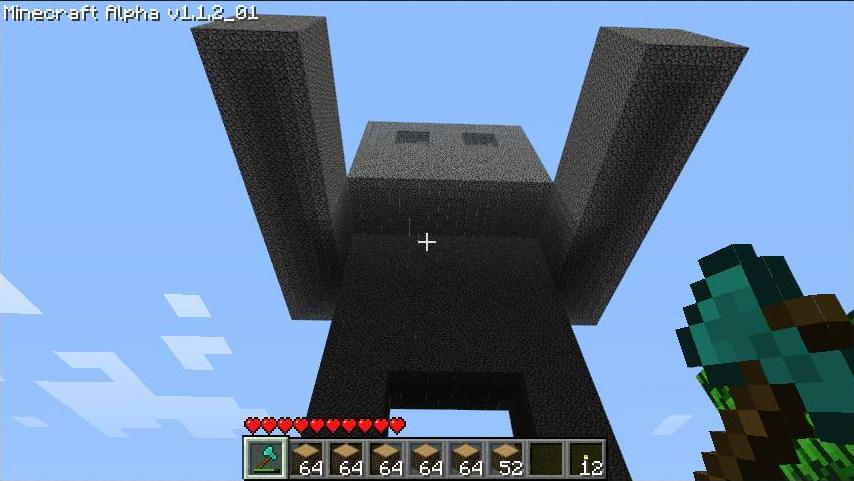This image is a detailed screenshot from the video game Minecraft, specifically from the Minecraft Alpha version 1.1.2-01, as indicated in white text on a blue sky background in the top left corner. The sky is a vibrant blue adorned with squarish white clouds. The main focus of the image is a towering, humanoid stone figure centrally positioned, composed of large blocky shapes. This figure has long, rectangular arms reaching towards the sky, a body, legs, and a square head featuring two slightly darker square eyes.

The perspective of the image suggests the viewer is positioned below, looking up at the imposing figure. To the right, there is a blocky tree-like structure with green and brown blocks, while in the bottom right corner, some blocky greenery and landscaping are visible.

Across the bottom of the image is a user interface displaying several hearts, indicating the health level, and a series of boxes showing the player's inventory. The first box holds an axe, while the subsequent ones are filled with items and numbers such as 64, 64, 64, 64, 64, 52, a blank square, and a 12, providing a glimpse into the resources available to the player. This screenshot encapsulates the quintessential blocky aesthetic and gameplay elements characteristic of early Minecraft versions.